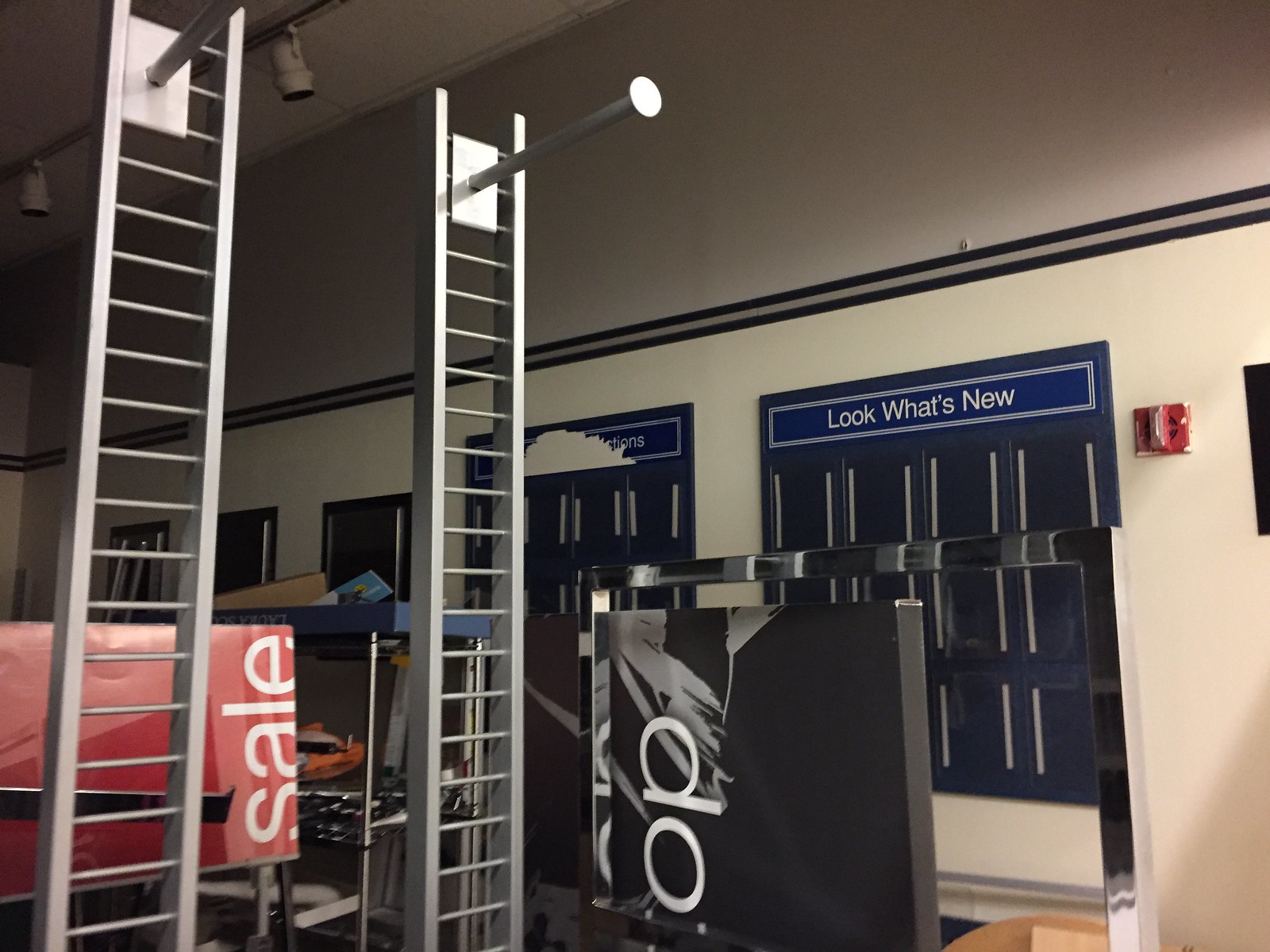This landscape photograph, in color, captures the interior of a high-ceilinged clothing store that appears to have been recently shut down. The room features white walls adorned with a black border halfway down, adding a frame-like effect. On the left side of the image, two upright silver racks stand, resembling small ladders with horizontal hanging rods ending in metal discs to prevent hangers from sliding off. Behind these racks, a red sign with white lettering that reads "SAIL" is visible at the very bottom, in addition to a tilted black sign displaying the incomplete letters "D.O." On the back wall, a blue sign with white letters proclaims "LOOK WHAT'S NEW" above areas where racks previously hung. The right side of the image reveals a red fire alarm and hints of other silver racks and equipment scattered in the background. The ceiling is supported by beams with large, unlit lights attached. Overall, the store looks barren with no merchandise, suggesting it has either been emptied out or is in the midst of a transition phase.